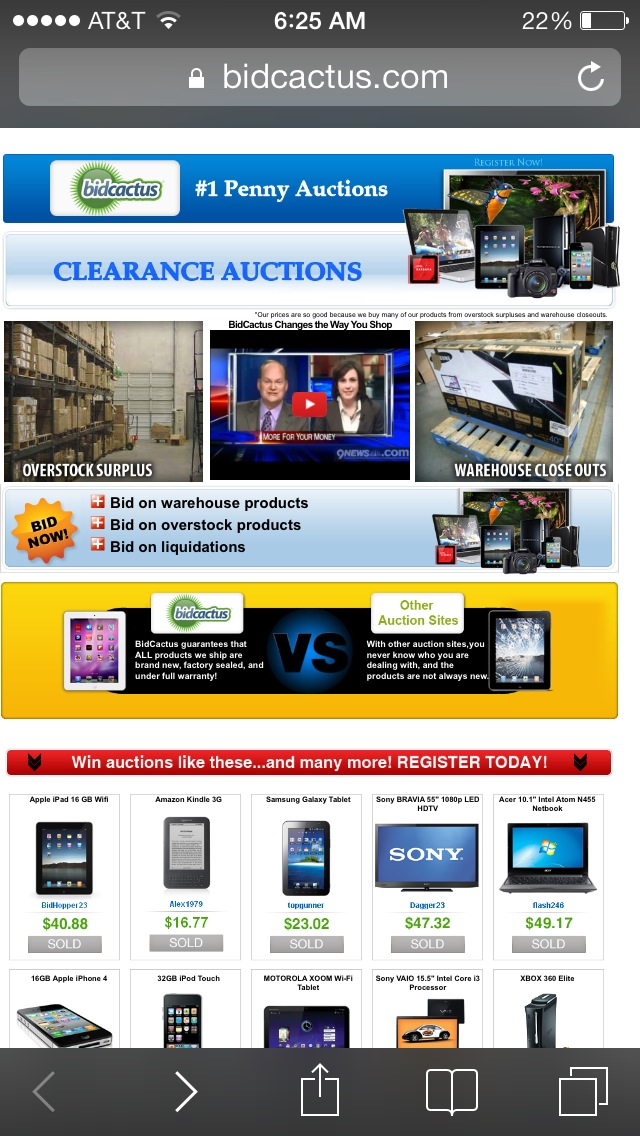This is a detailed screenshot of a mobile device displaying a webpage from BidCactus.com, captured at 6:25 AM with AT&T as the provider. The battery indicator shows a 22% charge. The website, branded as BidCactus, highlights itself as the "number one penny auctions" destination and promotes "clearance auctions." The page is filled with images of various electronics like TVs, iPads, iPhones, and other gadgets. Right below the headline, there are photographs of bulk warehouse items, including overstock and surplus products. A featured YouTube video of two individuals from 9newsstation.com adds a multimedia element.

The site encourages users to "bid now" on warehouse products, overstock products, and liquidation items, detailed next to an orange "bid now" icon. It boasts a guarantee that all products are brand new, factory sealed, and under full warranty, contrasting this assurance with the uncertainty associated with other auction sites. Additional visuals depict a range of electronics with prices, implying past sales and reinforcing the efficacy of the auction model. The bottom of the screen includes navigational icons for more browsing options. Overall, the screenshot portrays BidCactus as a dynamic auction site emphasizing quality assurance and a wide array of electronic products available through various bidding categories.